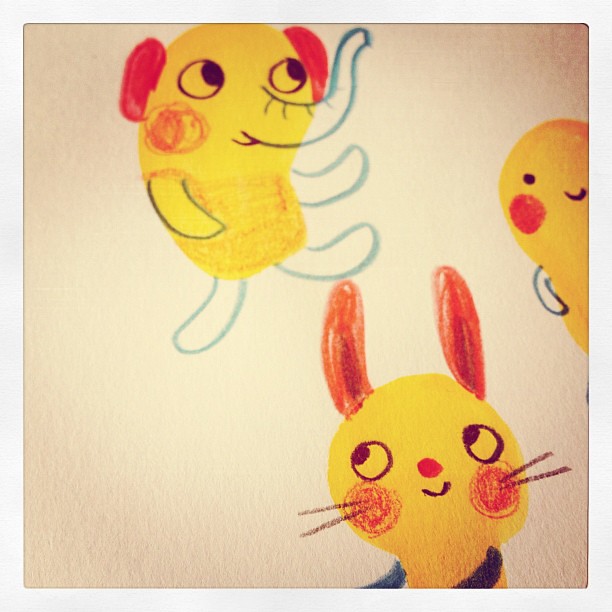This is a photograph of a whimsical, hand-drawn cartoon illustration that appears to be from a children's book or similar artwork. In the upper left quadrant, there is an elephant character, creatively constructed from a yellow bean-shaped body. This elephant features detailed black crayon drawings adding legs, arms, a distinct trunk, red ears, and prominent circular eyes with red cheeks, indicative of a playful, childlike style. In the bottom right corner, a large yellow shape has been transformed into a bunny-like figure, adorned with expressive big eyes, red cheeks, whiskers, and characteristic bunny ears. Additionally, in the upper right corner, there's another yellow bean shape, partially extending out of the frame, sporting a simple smile, a black dot for an eye, a red cheek, and a small arm. The colors predominantly consist of yellow, red, and black. The images, spread out across the page, appear to be created by an artist or author, likely intended for a children's book given the vibrant, engaging style and imaginative character designs.